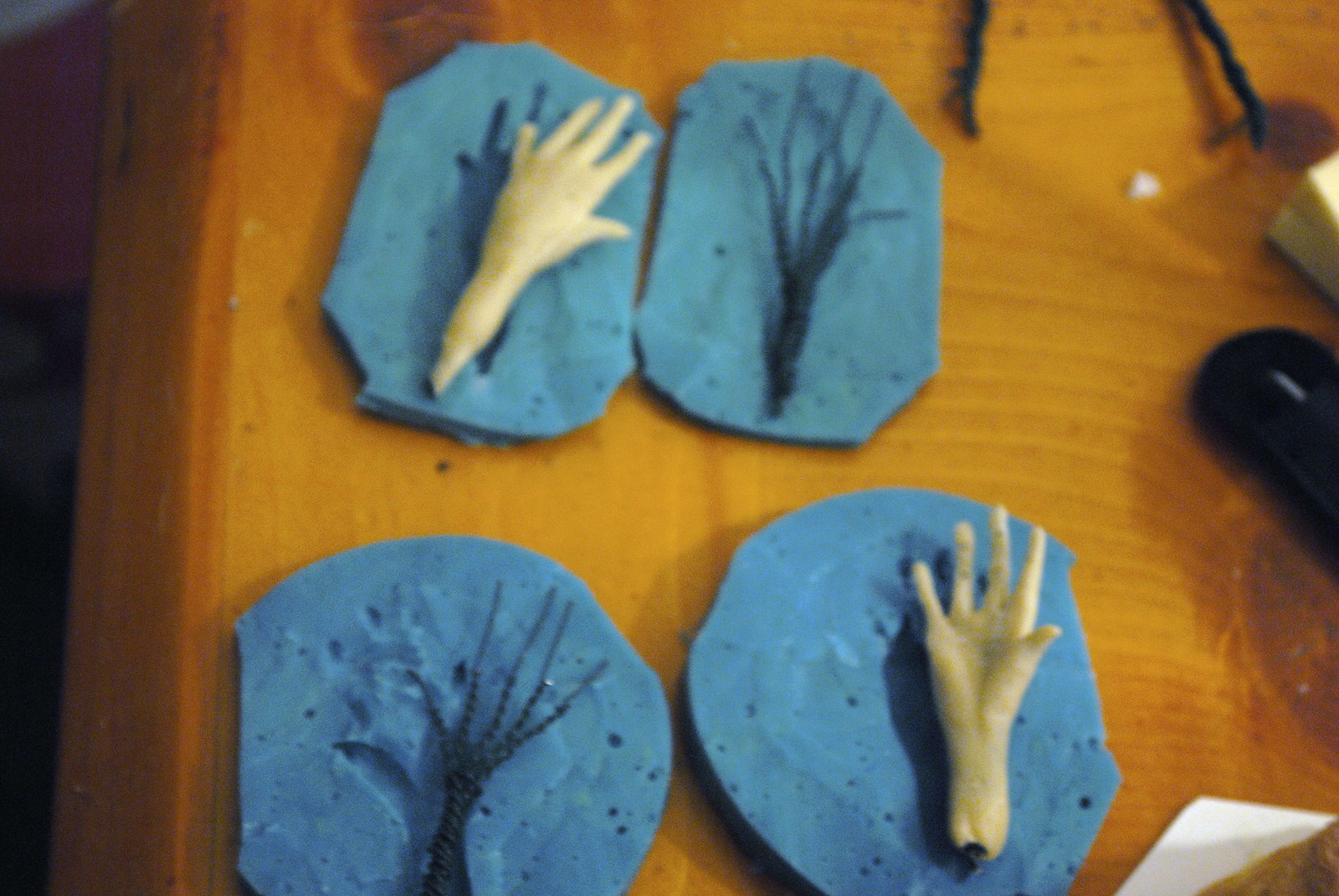The image shows a large wooden table, possibly made of oak or pine, with visible knots and wood grain patterns in an orange-brown hue. On the table, there are four round blue clay-like objects, arranged in a two-by-two stack. These blue clay molds each have imprints or features suggesting they were used to create hand shapes. Two of the blue molds contain white or waxy plastic hands, while the other two only display the hand-shaped indentations. Additionally, two black, stick-like objects, reminiscent of skeletal structures, are also present. The overall scene suggests an artistic or experimental setup, possibly for creating hand models, decorations, or Halloween props.